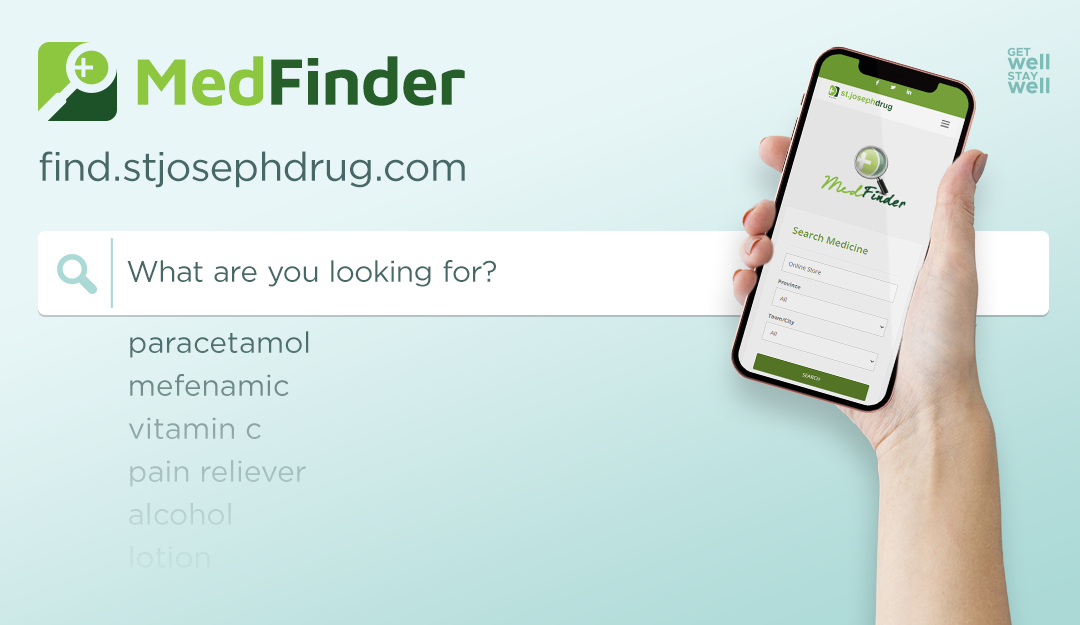A detailed photographic image portrays a web page primarily adorned in shades of light blue, green, and dark green, accentuated with white elements. Dominating the upper left corner of the page is a square logo featuring a green and dark green background with a white magnifying glass and a plus sign within it. Adjacent to this logo, "Med Finder" is prominently displayed in a sizable font, with "Med" in green and "Finder" in dark green.

The web address "find.stjosephdrug.com" is indicated below the title. On the right side of the image, a person is seen holding a mobile device with their right hand, showcasing fingers painted in red nail polish gripping the device. The screen of the mobile device is open to the Med Finder application, which mirrors the color scheme and logo of the web page. A search bar positioned at the top of the application interface prompts "What are you looking for" with an accompanying magnifying glass icon. 

Below the search bar, a list of keywords such as "paracetamol," "methamphetamine," "vitamin C," "pain reliever," "alcohol," and "lotion" is visible. To the right of the list, the encouraging message "Get well, stay well" is displayed.